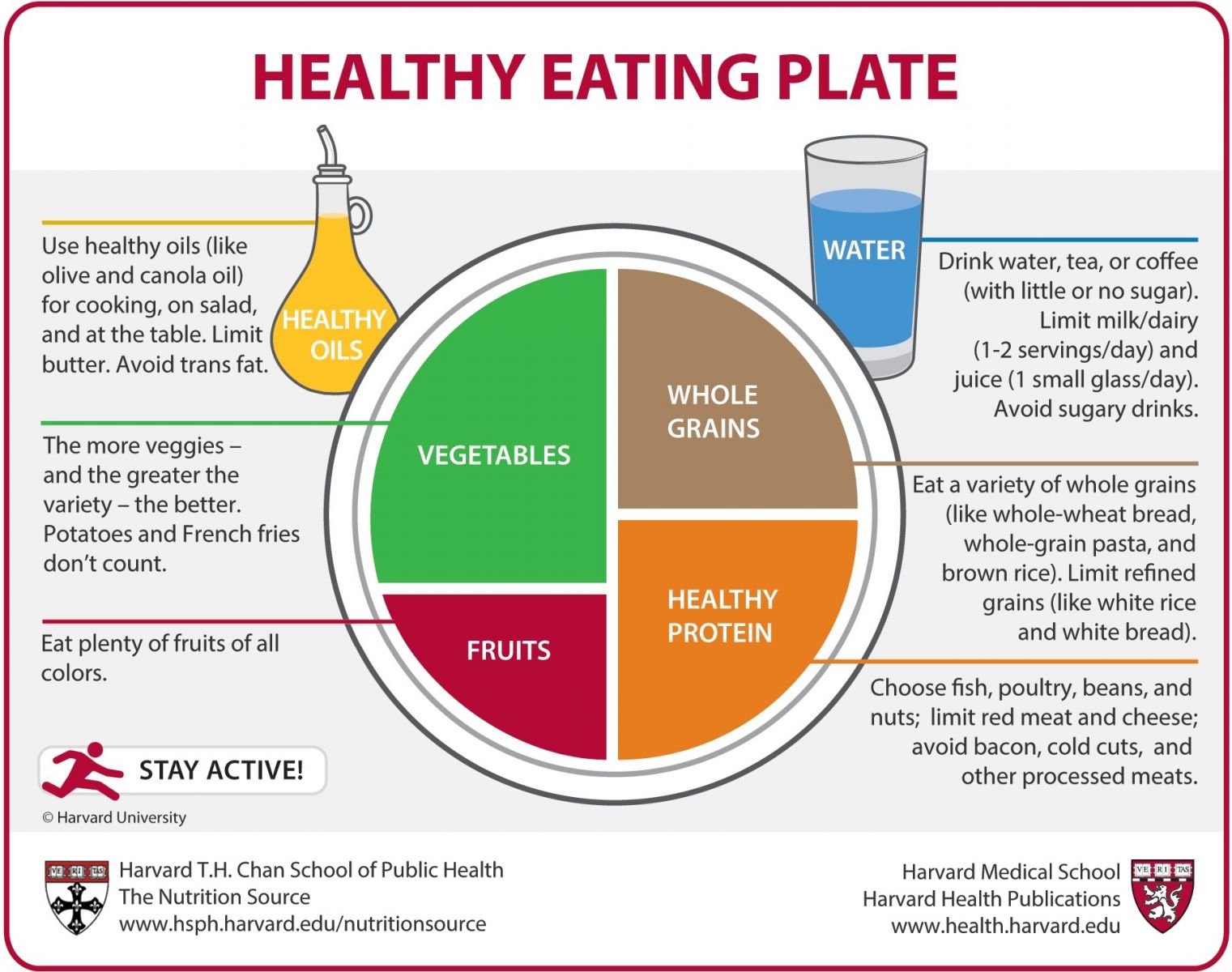The image displays a detailed "Healthy Eating Plate" that visually guides on how to proportion the different food groups for a balanced diet. According to the guidelines provided by Harvard Medical School, the plate should be divided as follows:

- **Fruits:** One-quarter of the plate should be filled with a variety of fruits. All types of fresh fruits are encouraged.
  
- **Vegetables:** Fill half of your plate with a diverse range of vegetables. Note that potatoes and French fries are not included in this recommendation.
  
- **Whole Grains:** Allocate one-quarter of the plate to whole grains. Suitable options include whole wheat bread, whole grain pasta, and brown rice. Avoid refined grains such as white rice and white bread.
  
- **Healthy Protein:** Dedicate the remaining quarter of the plate to healthy proteins like fish, poultry, beans, and nuts. It is recommended to limit the intake of red meat and cheese and to avoid processed meats like bacon and cold cuts.

The plate also includes guidance on oils and fats, recommending the use of healthy oils like olive oil and canola oil for cooking, dressing salads, and adding to food at the table. It suggests limiting the use of butter and completely avoiding trans fats.

In terms of beverages, it advises drinking water, tea, or coffee and to limit dairy and juice intake. Sugary drinks should be avoided entirely.

This comprehensive guideline aims to promote a balanced diet that supports better health and well-being.